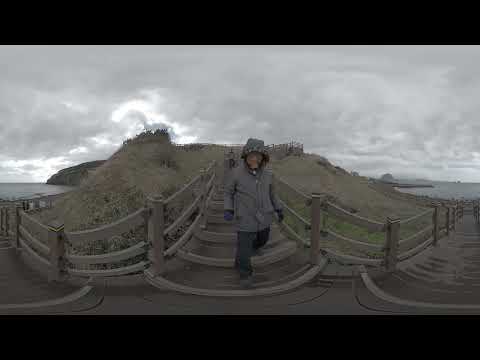The image captures a dramatic, overcast sky, densely packed with clouds that allow minimal light to pass through, casting the landscape in muted colors. At the center of the image stands a figure, possibly a person, enveloped in ambiguity due to the indistinct features that lend a mysterious quality. This central figure is accompanied by a curious blue patchy area beneath them, the nature of which is unclear but suggests it could either be an artifact of the image or an actual object like a tent. Surrounding this figure is a sweeping landscape defined by varied terrain. To the left, the land inclines, sweeping down into a valley shrouded in darkness, giving way to bodies of water on both sides. To the right of the figure, the land again slopes down towards a lake, bordered distantly by a small mountain that merges with the horizon. A prominent, man-made fence with large poles is visible to the left and right of the figure, adding to the scene's enigmatic charm. The background features tall, wavy trees standing atop a large mound, contributing to the overall sense of a dense, outdoor setting. The ground beneath the figure is thatched and appears beaten down, indicative of a rugged, well-trodden environment viewed as though from an island's perspective, possibly using panoramic imaging.